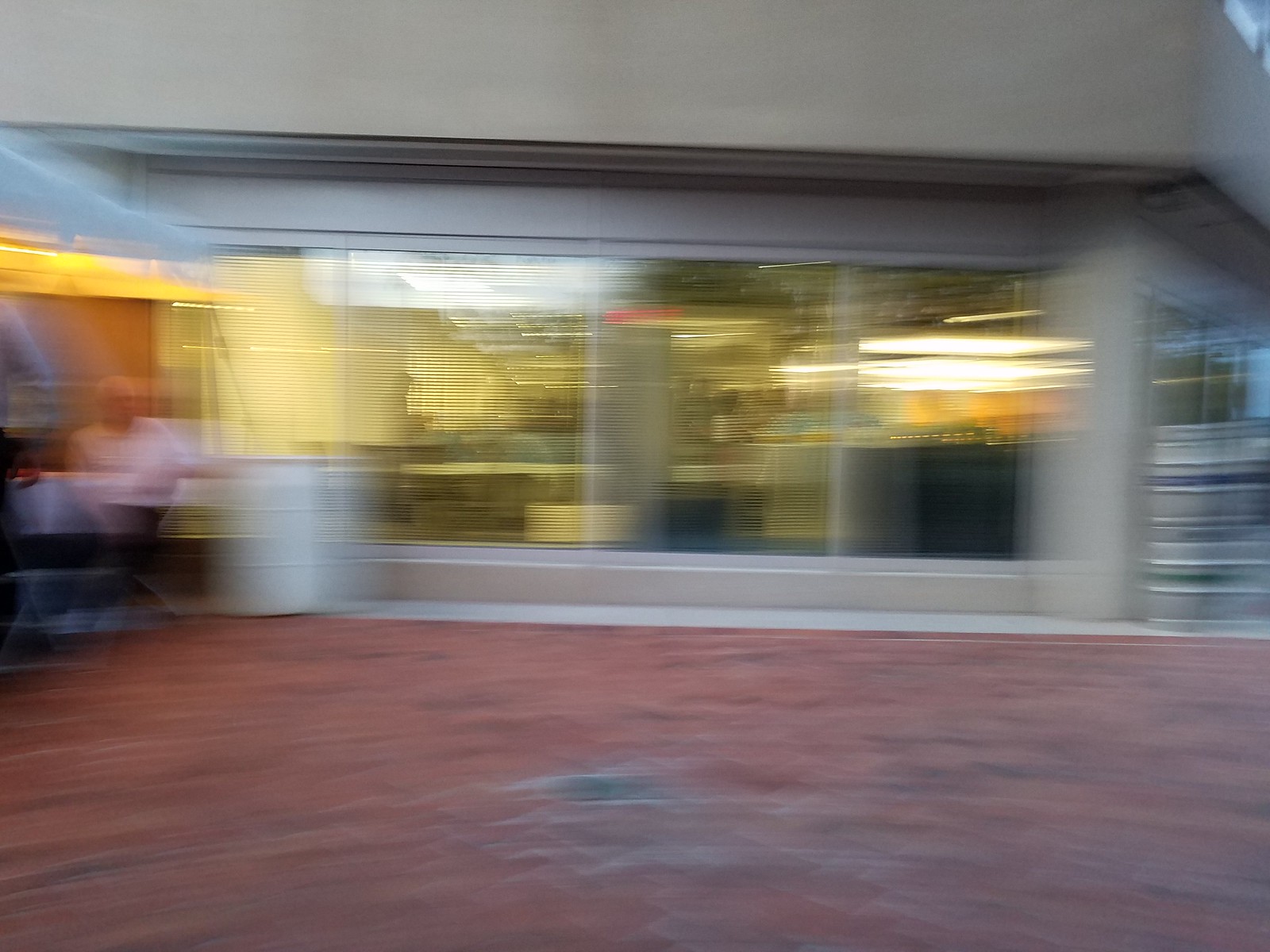This outdoor photograph, though very blurry, reveals the facade of a building with large windows featuring open blinds. The structure appears to be an office, given the size and arrangement of the windows. To the left, an indistinct figure of an older man can be observed; he is dressed in a white shirt and dark pants. The ground beneath the windows has a reddish hue, possibly indicating a red brick surface. The building's exterior extends upwards with what seems to be a stucco finish, although the blur obscures finer details. On the right side of the image, there is an unclear silver and black object, marked with streaks, whose purpose and form remain indiscernible.